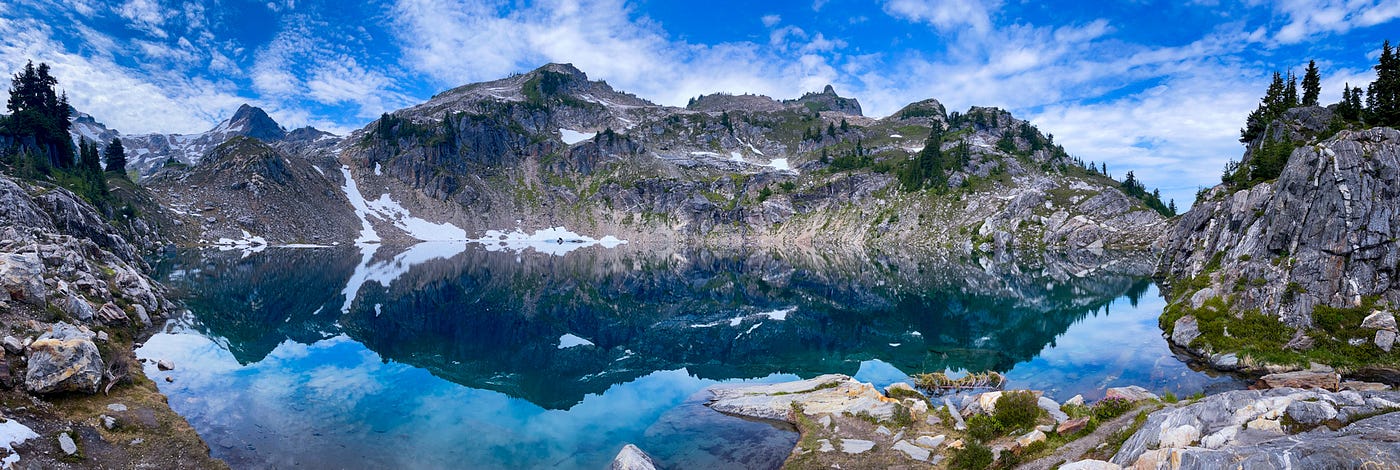The image is a stunning, panoramic view of a vast natural landscape showcasing a vivid blue sky dotted with scattered white clouds, reflected flawlessly in a crystal-clear glacier pool. Framing the background are majestic mountains, characterized by their rocky, stone texture and sporadic patches of snow. These mountains stretch into the distance, featuring both tall cliffs and smaller boulders, with hints of moss and sparse vegetation such as pine trees, especially towards the left side of the image. There is a clear visual contrast between the moss-covered stones and the serene, blue pool, which mirrors the sky and the towering peaks above. At the forefront, there are some bushes and moss, suggesting a path leading into the tranquil water, which allows the entire scenery to appear almost surreal with its pristine reflection and vibrant natural elements.